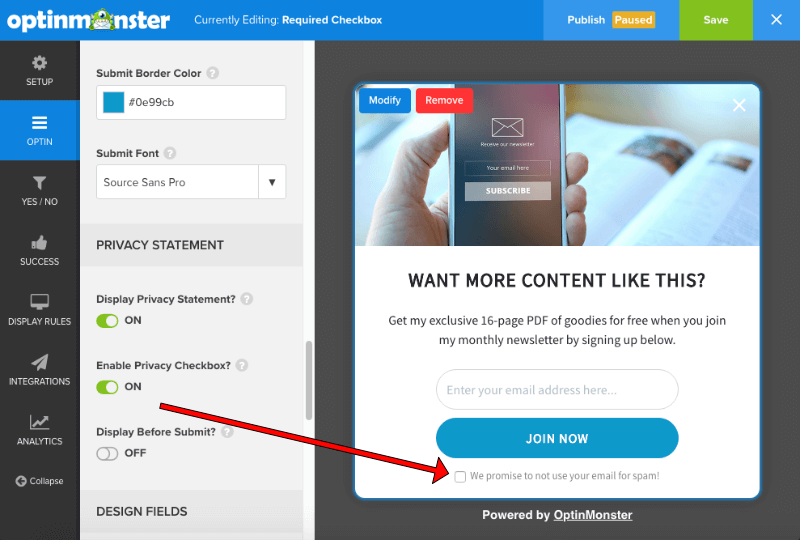In the screenshot of the OptinMonster website, we're observing the setup interface for creating an opt-in or landing page. Dominating the right side of the image is the landing page preview, outlined with a dark gray background. Prominently displayed on this page is a red arrow pointing to a clickable box that reassures users with the text, "We promise to not use your email for spam." The OptinMonster logo is easily visible in the top left corner of the interface.

On the left side of the screen, a menu offers various tabs, including Setup, Opt-in, Filtering, Successes, Display Rules, Integrations, and Analytics. The Opt-in tab is currently active, allowing users to customize elements such as the border color, font, and privacy statements for the page. Options within this menu include toggling the privacy statement and privacy checkbox on or off, providing further personalization and assurance for potential subscribers.